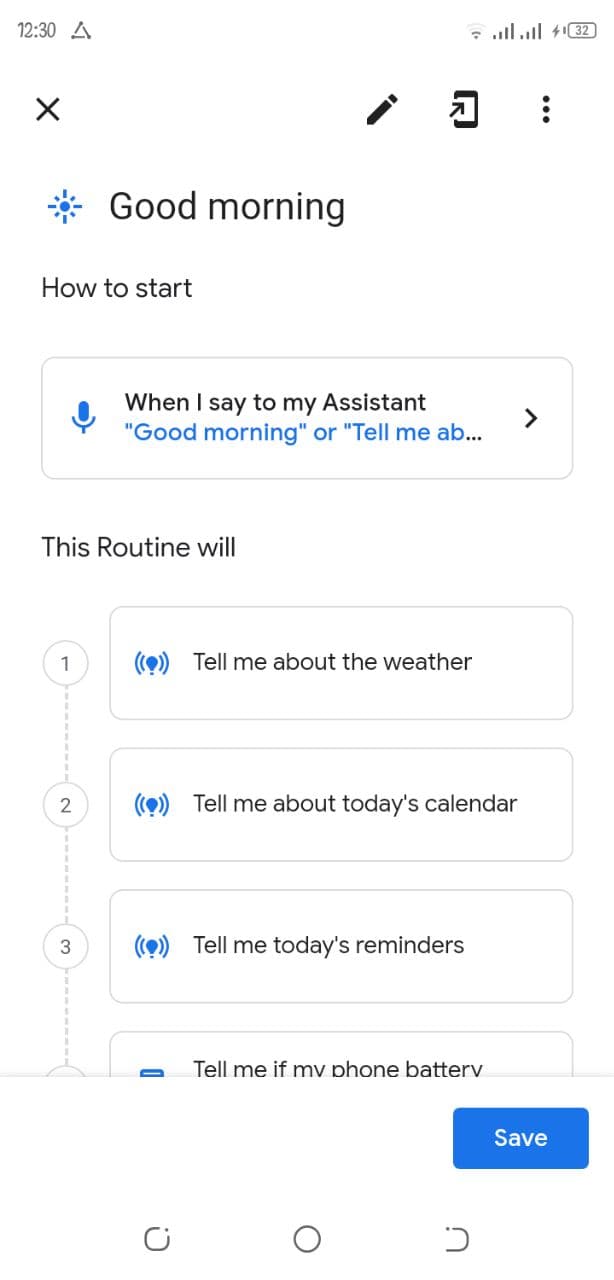This is a detailed screenshot from a person's smartphone screen. In the top left corner, the time is displayed as 12:30. In the top right corner, there are icons indicating Wi-Fi connectivity, cellular coverage, and a battery level at 32%. Below these are several icons: a black "X," a black pencil icon, a black smartphone icon, and a column of three vertical black dots.  

Centered on the screen is a blue, sunburst-styled icon with the text "Good Morning" followed by subtitle text that reads: "How to start. When I say to my assistant, 'Good Morning,' or 'Tell me A B...' This routine will: 1. Tell me about the weather. 2. Tell me about today's calendar. 3. Tell me today's reminders. 4. Tell me if my phone battery..." The text is cut off at this point, leaving the remainder of the list obscured from view.  

Beneath this text block is a prominent blue rectangle with white text that says "Save," which is centered on the screen. The image is strictly a screenshot of a mobile interface—it does not contain any photographic elements such as people, animals, birds, fish, or plants. The emphasis is entirely on the text and icons described.